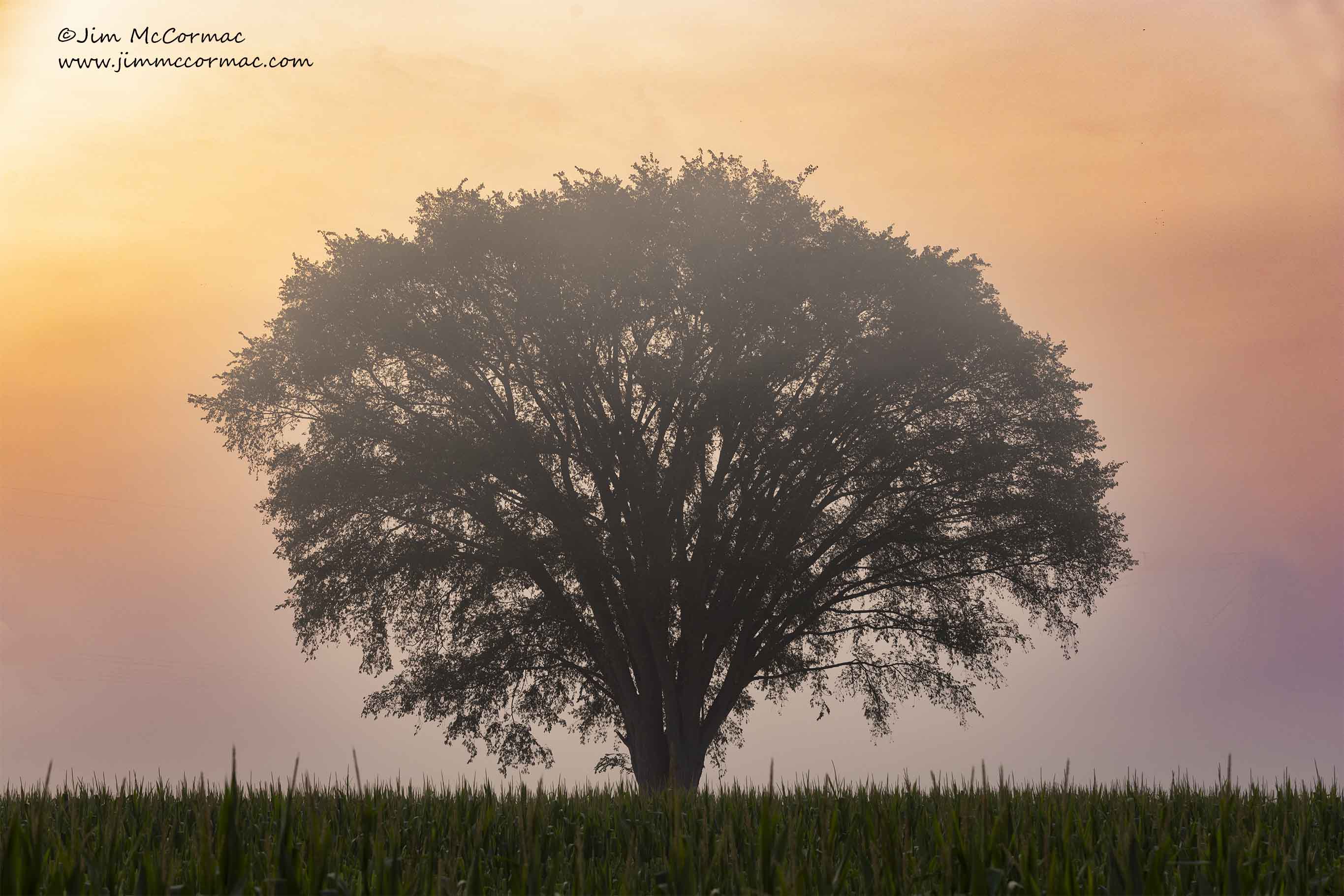This is a painting of a lone tree standing in an otherwise empty field, set against the vibrant colors of a dusk sky. The tree, situated at the center and serving as the focal point, appears shadowy and dark, almost blending into the green grass that spreads across the foreground. The sky above features a stunning gradient of colors, with hues transitioning from orange and pink to purple, white, and blue, suggesting the serene beauty of sunset. In the upper left-hand corner, sunlight peeks through subtly, and a black calligraphy font marks the copyright text, "Jim McCormick," along with the website "www.jimmccormick.com." The image is a striking capture of nature’s tranquil yet vivid display as day turns to night.